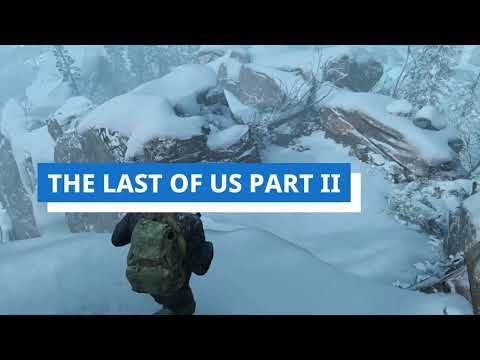In the image, we observe a screenshot from the video game "The Last of Us Part 2." The scene presented follows a third-person perspective of the character Abby, who appears centered yet slightly to the left. She is trekking down a snow-covered hill, adorned in a dark, long-sleeved outfit and carrying a stuffed, camo-green backpack. The character’s head isn’t clearly visible. The top 10-15% and the bottom 10-15% of the image are letterboxed with black bars, creating a square format. 

The game’s title, "The Last of Us Part 2," is prominently displayed in bold, white sans-serif text within a blue rectangular banner at the top of the screen. This blue banner is echoed by a white rectangular background at the bottom right, reinforcing the title's presence. 

The environment is strikingly wintery, with fluffy layers of white snow blanketing the hill and extending down to descending cliffs. A few wiry, barren trees stand scattered in the distance, also covered in snow, contributing to the desolate and cold atmosphere. The colors featured in the image include various shades of white, gray, green, black, blue, and brown, highlighting the stark, wintry landscape against Abby’s darker attire. The composition emphasizes the vastness of the snowy terrain, with Abby as the focal point of her isolated journey.